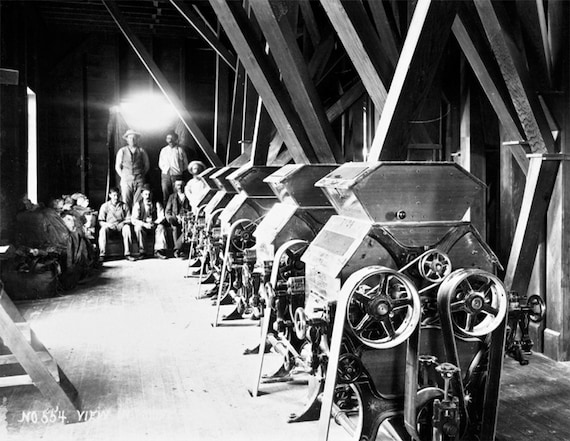In this black and white photograph, we see an industrial scene set inside a wooden structure that resembles a barn. Dominating the image are five silver metal machines lined up in a row, each equipped with circular wheels on their sides. The purpose of these machines is not immediately clear, though they appear to be involved in processing tasks, possibly grains or wheat. The background is illuminated by a vibrant white light, shining prominently and drawing the viewer's eye. Additionally, six men are positioned in the back of the room—two standing and four sitting—all intently facing forward, seemingly observing the machinery or possibly posing for the photograph. Some details in the lower left corner of the image include white text, though it is not legible. This photograph captures a moment of industrialization with an air of mystery about the function and focus of the gathering.